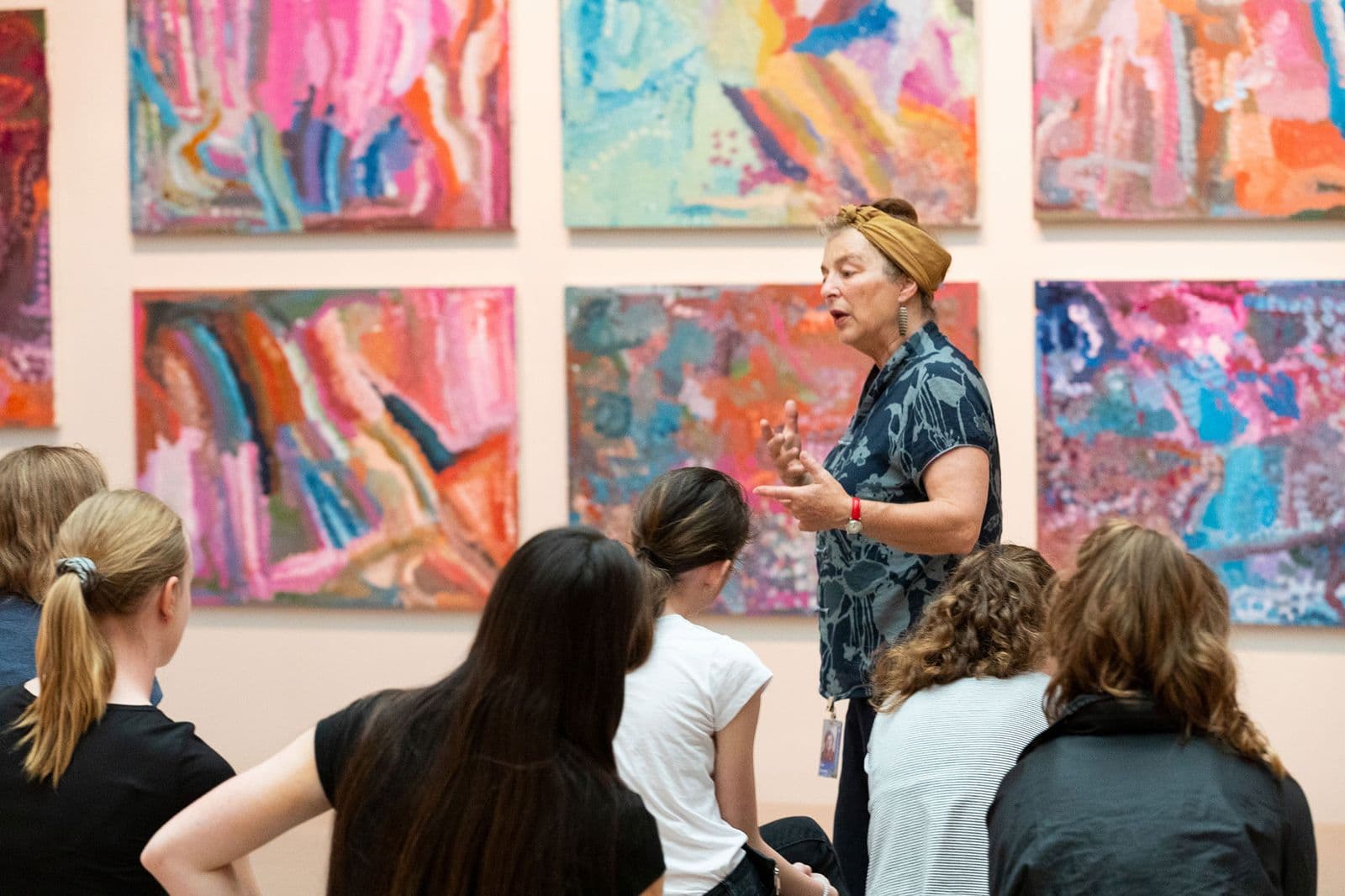In an indoor classroom setting with a peach-colored wall adorned with several vibrant, abstract paintings in shades of pink, blue, orange, and white, a mature art teacher stands engaging a group of six young female students seated in front of her. The teacher, dressed in a loose gray blouse with a black and green shirt and sporting a beige scarf around her head, gestures animatedly as she speaks. Her hands are outstretched and she wears a red wristwatch, with an ID tag clipped to the bottom right of her shirt. The abstract artworks behind her are geometric and colorful, devoid of discernible shapes, adding a creative backdrop to her lesson. The girls, dressed casually in t-shirts and jackets, are focused on the teacher, who is passionately explaining the fundamentals of art with paint and brushes.